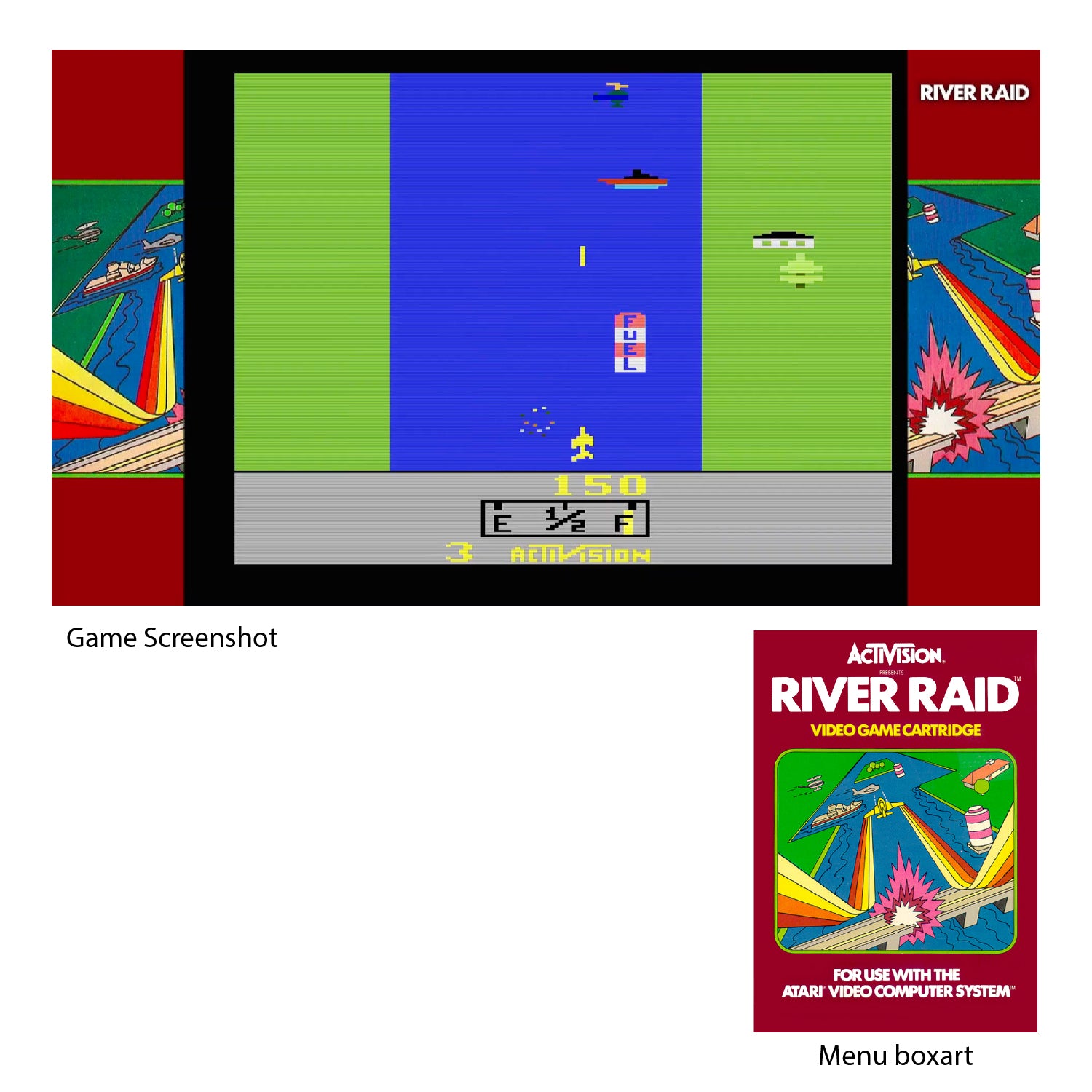This image features the box art and a gameplay screenshot for the "Activision River Raid" video game cartridge, designed for the Atari video computer system. The box art is prominently displayed in the lower right corner with a vibrant red background and eye-catching, brightly colored graphics that depict a portion of the game's action. "Activision River Raid video game cartridge for use with the Atari video computer system" is clearly written on the box. The gameplay screenshot covers the upper portion of the image, displaying a detailed scene. The primary gaming area is divided vertically into three sections: two green strips on the sides represent land, while a central blue strip symbolizes a river. Integral game elements are illustrated, including a rocket ship, boats, fuel indicators, a tank, and a helicopter, and the player's score of 150 points is highlighted in yellow at the bottom center. The background outside the gaming screen consists of a mix of blood-red and beige-brown hues with additional graphics. The image is framed with text that includes "menu BOX ART," emphasizing the box art depicted below the gameplay screenshot. The intricate design and vividly detailed visuals communicate the dynamic and interactive nature of the game.